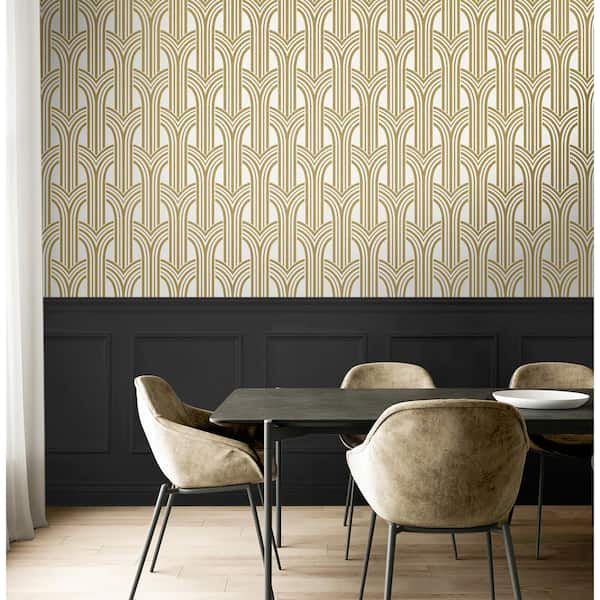The image depicts a modest dining room characterized by a black table with gray metallic legs, positioned centrally on a light brown hardwood floor. Four cup-shaped chairs, covered entirely in gray fabric, are arranged around the table, which seems to have a foldable, practical design rather than a permanent, ornate one.

The walls present a distinct dual-tone aesthetic: the lower half is adorned with dark black, square-patterned wainscoting, while the upper half features a white wallpaper embellished with overlapping light gold arcs. On the far left side, diaphanous white curtains hang from ceiling to floor, allowing light to filter through, creating a delicate contrast with the darker elements in the room. Overall, the dining area combines simplicity with subtle decorative elements, offering a cozy yet unpretentious atmosphere.